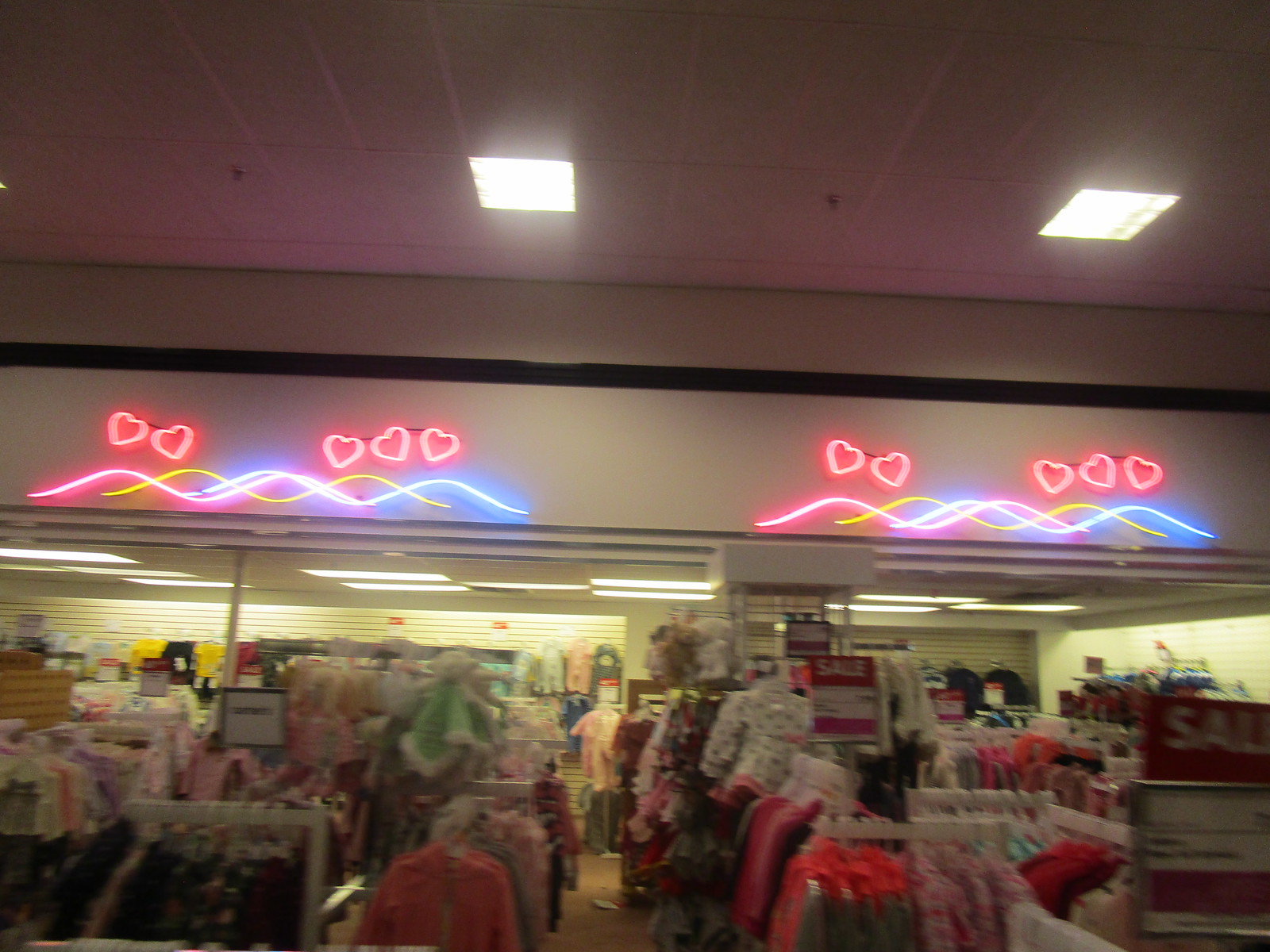The image depicts a section of a clothing store, likely taken at night, evidenced by the overall dim lighting pierced only by square fluorescent ceiling lights—one centrally located and another to the right. The back wall captivates attention with its decor, featuring 10 neon red heart shapes and a series of colorful waves in pink, yellow, and blue. The colorful display illuminates racks of clothing below, which are neatly arranged. On the left, the racks hold a variety of shirts, coats, and jean jackets, while on the right, there are more jackets, including black leather ones, prominently marked with sale signs. In the middle of the scene, a red sale sign stands out amidst the vibrant clothing collection, suggesting targeted promotions. The store appears to cater to a wide age range, with clothing for women and possibly girls aged 8 and up. Despite the busy arrangement of clothes and sale signs, the colorful neon hearts and waves create a focal point in this lively snapshot of a department store's shopping area.